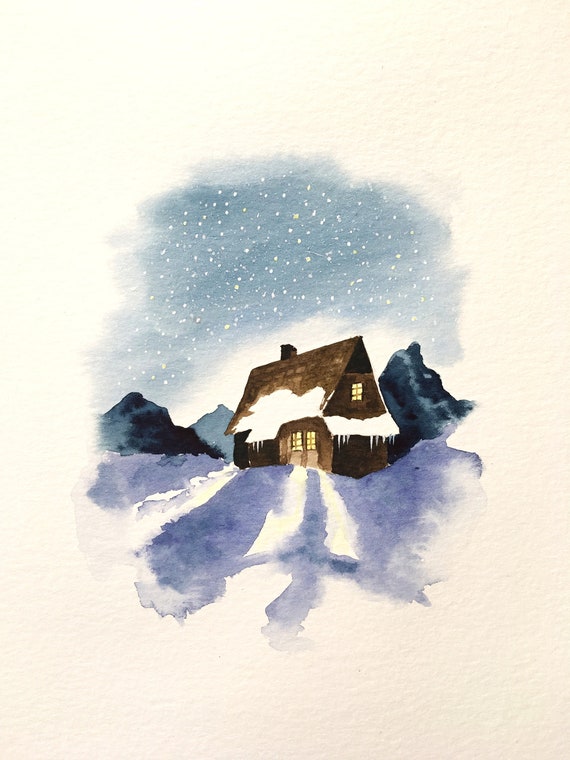This detailed painting, resembling a watercolor, showcases a snowy and serene nighttime scene featuring an isolated, dark brown A-frame cabin with a tall, triangular shingle-thatched roof partially covered in snow and icicles hanging from the sides. Light warmly emanates from two large doors and a smaller attic window on the top right, casting a gentle glow against the icy blue and white hues of the surroundings. The ground and the middle area of the roof are blanketed with snow, with patches of dark blue reflecting the starry sky. The scene is framed by dark green trees on either side of the cabin, and further back, jagged navy blue mountains rise against the grayish-blue sky where delicate snowflakes dot the air. A chimney suggests a cozy fireplace within, adding to the tranquil and inviting atmosphere of this small, yet bright refuge amidst the snowy wilderness.